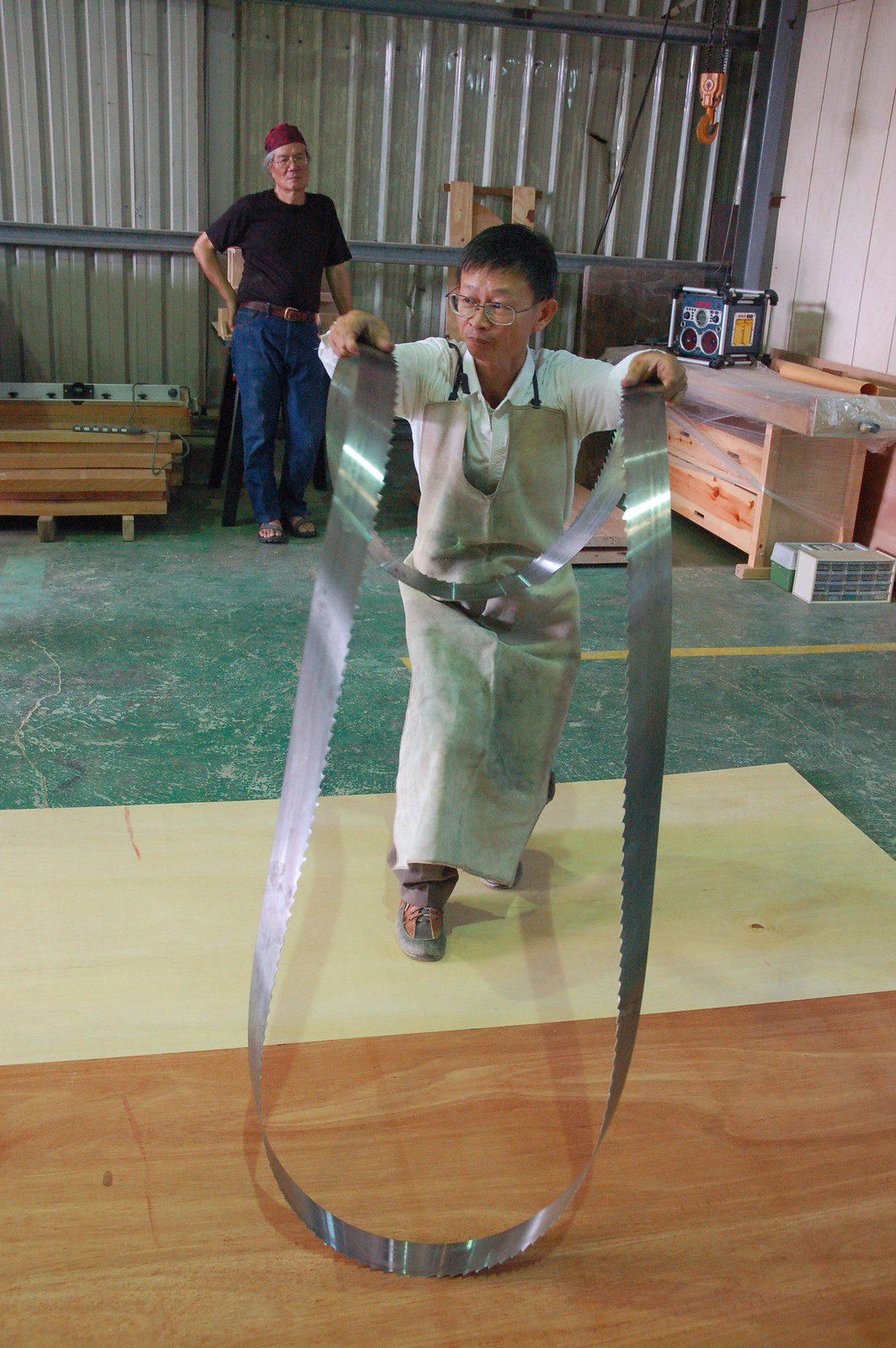In this image, we see two Asian men in what appears to be a large, industrial garage or studio with a corrugated metal wall and stained concrete floor. The space is expansive, likely reaching two stories in height. The man in the foreground, who appears to be in his 50s or 60s, wears wire-rimmed glasses, a long beige apron that reaches his ankles, a white t-shirt, brownish pants, and orange and black tennis shoes. He is holding a giant piece of curved, sawtooth-edged metal with both hands, which spans approximately 20 feet if laid out flat but appears circular and reminiscent of a shark’s jaw when flopped over in his grip. The ground near him shifts from beige and brown wooden surfaces to a green marble section, dusted and marked with a yellow strip. In the background stands another older man with black hair, glasses, a red hat, a black shirt, blue jeans, and black sandals, one hand positioned thoughtfully on his hip as he observes the scene, suggesting that they are on the verge of starting a project involving the metallic object.